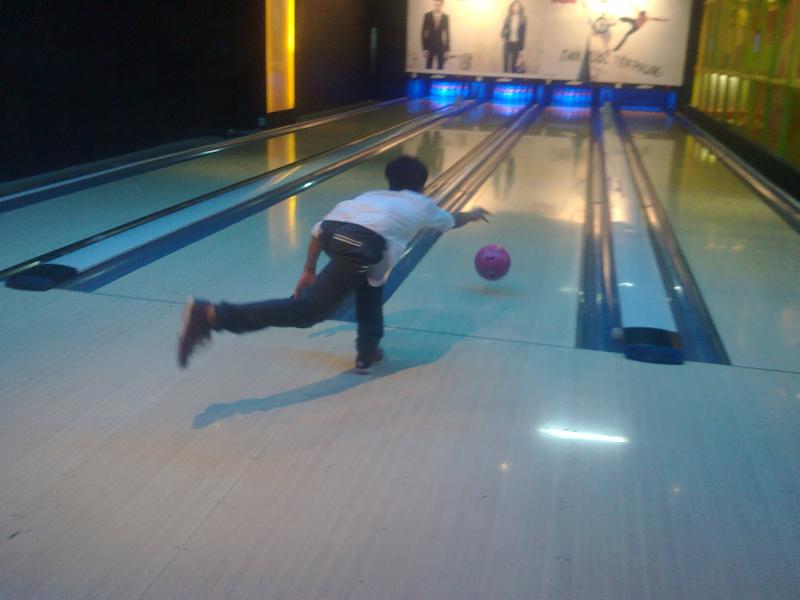This detailed photograph captures the dynamic moment of a person bowling inside a four-lane bowling alley. The scene is set in the third lane from the left, where a bowler with dark hair, dressed in a white shirt and blue pants, is in mid-motion. The individual is just releasing a dark pink bowling ball, with their right leg extended into the air and their left leg firmly planted on the ground. Adding to the intrigue, the bowler sports a fanny pack or similar accessory around their waist.

The lanes are clearly divided by gutters, guiding the eye towards the glowing blue pins with purple stripes at the end of the alley. In the background, above the pins, are three distinct images that could potentially be advertisements: one appears to show a man in a suit, another seems to depict a woman in a dark jacket over a white top, and the third, although blurry, suggests the outline of a human figure. The atmosphere is vividly captured, highlighting both the action in the foreground and the intriguing visual details in the background.